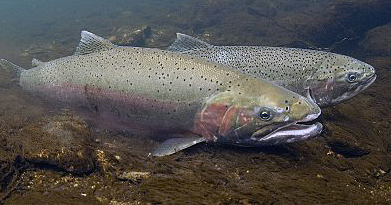This landscape photograph captures an underwater scene featuring two large, grayish-green fish, each adorned with numerous black speckles on their bodies. The fish dominate the center of the image, giving a close-up view of their physical features and the clear water surrounding them. The larger fish in the foreground displays an open mouth and visible right fin, outlined against the faintly visible brownish seabed, giving the impression of a natural, undisturbed habitat. Its body exhibits a blend of greenish-gray tones with an orange tinge around the gills and distinctive speckling along its top. The second fish, partly obscured by the first, shows a slightly darker gray with more pronounced speckles and its mouth remains closed, adding to the serene yet intense atmosphere of the scene. The backdrop of the image suggests the ocean floor, replete with rocks and covered in a layer of moss, dust, and mud, creating a well-lit and natural underwater environment.